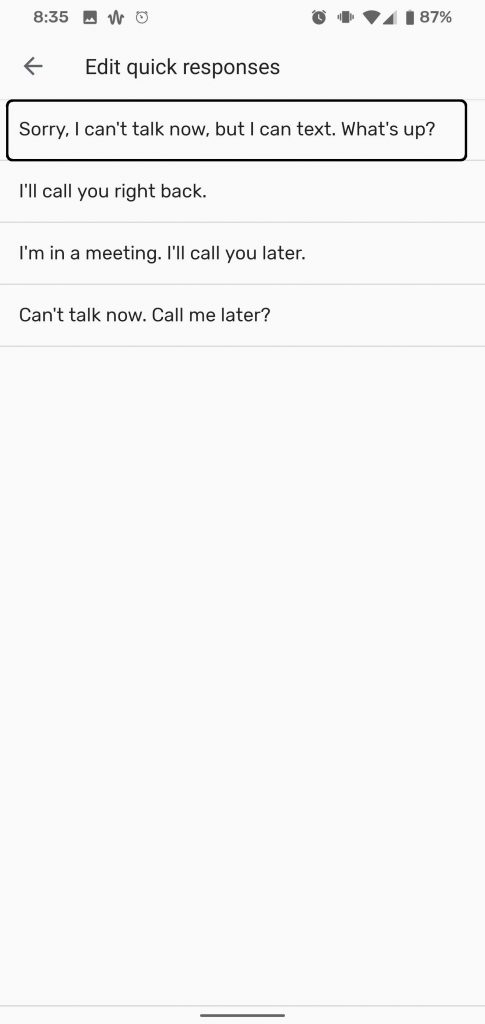The image showcases a mobile interface designed for quick text responses. At the top of the interface, the current time is displayed as 8:35. Adjacent to the time are several icons: a thumbnail picture, a heart rate symbol, an alarm clock, a buzzing phone icon, a WiFi indicator, and the battery level at 87%.

Below these elements, there is a section labeled "Edit Quick Responses," highlighted by a black box indicating it is currently selected. This feature allows users to send pre-scripted messages when they are unable to type out a response. The following quick response options are visible:

1. "Sorry, I can't talk now, but can I text what's up?"
2. "Call you back."
3. "I'm in a meeting, I'll call you later."
4. "I can't talk now, call me later."

The interface background is either white or light gray, providing a clear and clean look against the black text. The left arrow icon at the top left of the screen allows users to navigate back to the previous menu.

The design is user-friendly, making it easy for anyone who is pressed for time to quickly select and send an appropriate response.